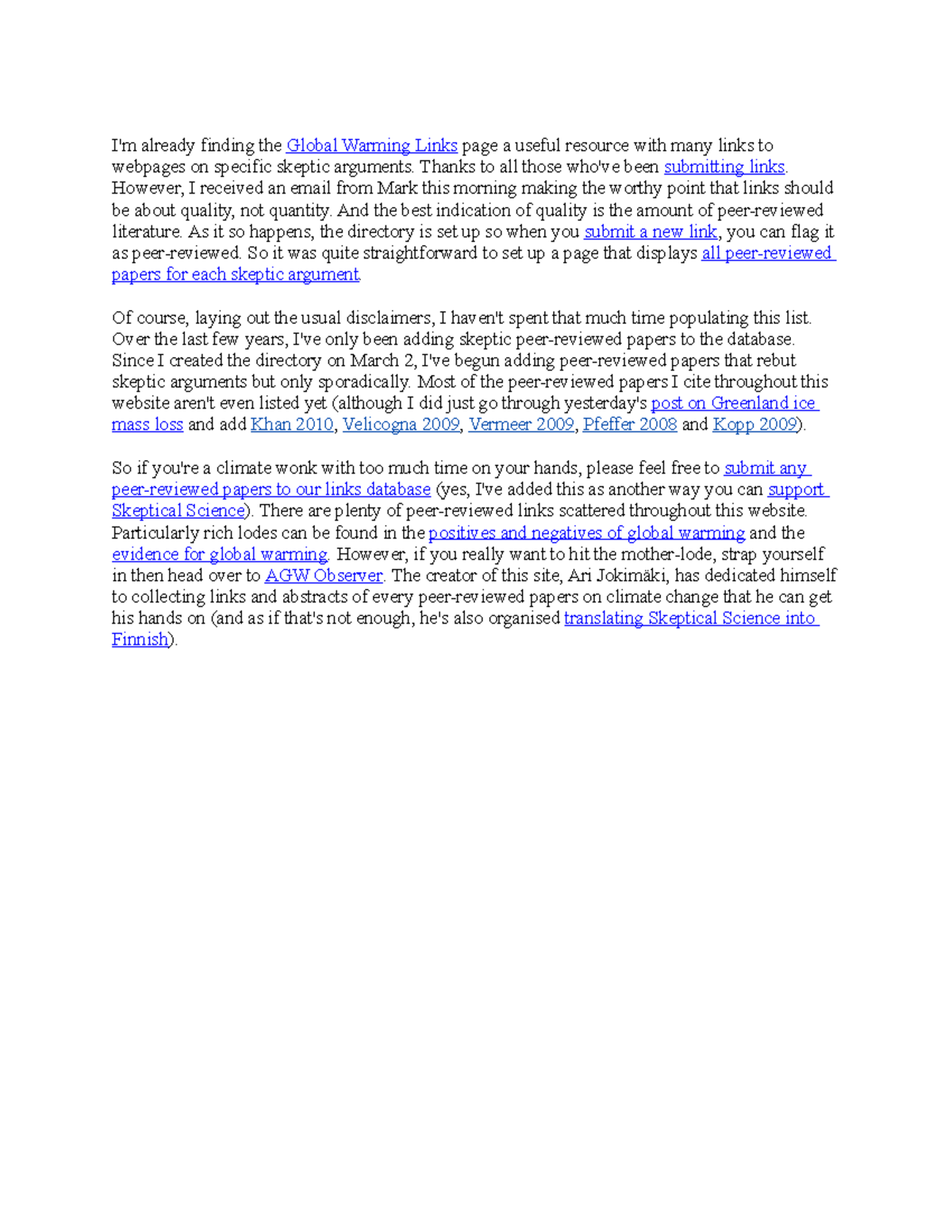The image contains three paragraphs of text, with several parts highlighted in blue and underlined. 

In the first paragraph, the text is written in very small font. Within this paragraph, certain phrases are emphasized in blue with blue underlines. The first highlighted phrase reads "global warming links," followed by "submitting links," and "submit a new link." The paragraph also includes a section that states "all peer-reviewed papers for each skeptic argument."

The second paragraph contains a description of a post titled "post on Greenland ice mass loss," which is also highlighted in blue with a blue underline. Further down, there are references to specific years written in a lighter font, including "2010," "2009," "2008," and once again "2009."

In the third paragraph, the text instructs readers to "submit any peer-reviewed papers to our link database," with certain parts underlined in blue. Notable highlights in this paragraph include "underlying support," "skeptical science," "positives and negatives of global warming," "evidence of global warming," "AGW observer," and "translating skeptical science into Finnish."

Overall, the image appears to detail various links and references related to global warming, including peer-reviewed papers, posts on specific topics such as Greenland's ice loss, and information translated into Finnish.